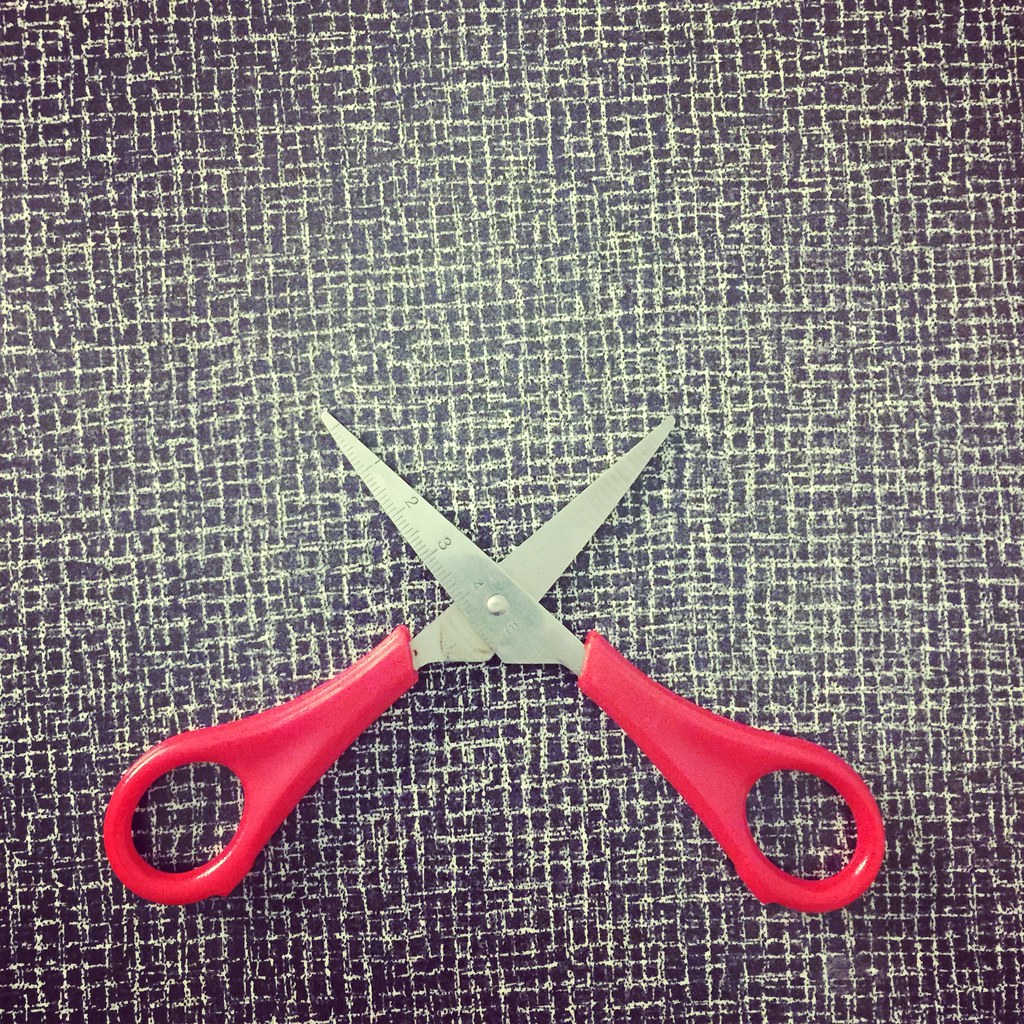This detailed color photograph depicts a small pair of sewing scissors prominently positioned against a textured fabric background. The scissors feature red plastic handles that exhibit a slight reflective quality, and their metal blades are fully open, forming an X-like shape. One of the blades is inscribed with a ruler marked from 1 to 5 inches, featuring tiny increments indicating measurements. The scissors' blades are short, riveted together at the center, and display a bit of dirt on one. The background material has a complex, textured appearance, resembling a cross-hatched pattern in black with interwoven white scratches or threads, creating a grid-like effect. The scissors are centrally placed on this fabric, making them the focal point of the image.